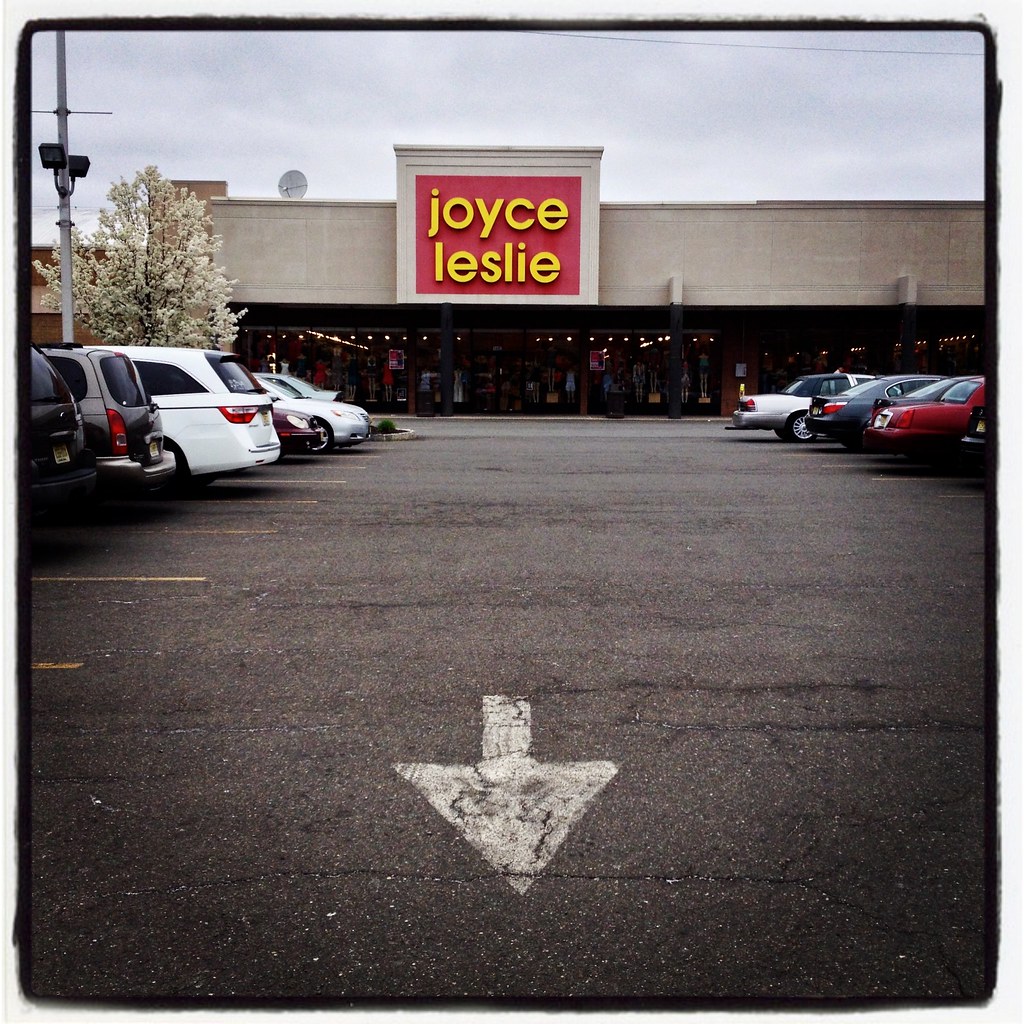The image depicts a parking lot leading up to a department store named Joyce Leslie. The department store features a glass front with a wide, concrete-colored top. The store's sign is rectangular, painted in red with lowercase yellow lettering that spells "Joyce Leslie." The parking lot, made of asphalt, consists of perpendicular spaces lining a one-way street, which is somewhat unusual since perpendicular parking lots typically accommodate two-way traffic. The scene suggests a relatively recent period; despite the presence of some older cars, there are also modern-looking vans. The weather appears to have been rainy, potentially during springtime, as indicated by a blooming dogwood tree to the left of the store. The interior of the store is not visible due to darkened glass, though some lights are discernible along the roofline.